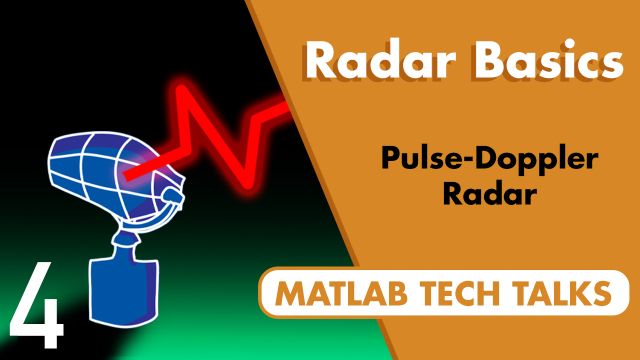The image is a detailed advertisement or poster for MATLAB Tech Talks, specifically featuring a segment on "Radar Basics" and "Pulse-Doppler Radar." The left side of the image showcases an illustrated radar gun in blue and white, set against a gradient background that transitions from dark green at the top to lighter green near the bottom. Emerging from the radar gun is a red zigzag line symbolizing a signal or pulse. Adjacent to the radar gun is a large, white number "4." The right side of the image displays text in black and white over a beige or orange background. The text reads: "Radar Basics," "Pulse-Doppler Radar," and at the far bottom, encased in a small white box with light brown lettering, it reads "MATLAB Tech Talks."